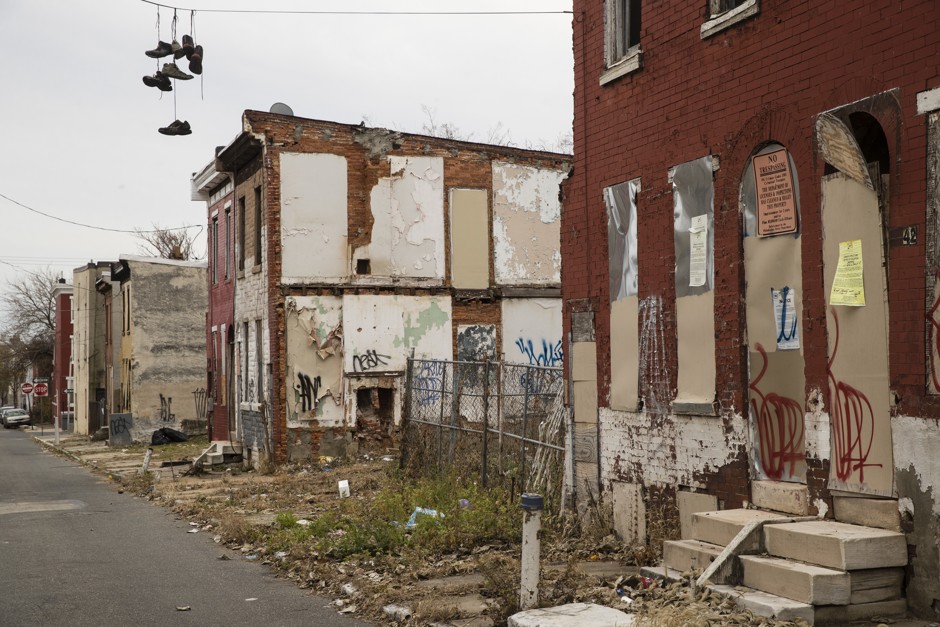The photograph showcases a dilapidated, abandoned urban neighborhood under a gray-blue sky. Dominated by red-orange brick buildings, the scene is characterized by neglect and decay. The structures, many with boarded or broken windows and doors haphazardly sealed with cardboard, display signs of long-term abandonment. "Condemned" and "No Trespassing" signs are visible, reinforcing the sense of desolation. The sidewalks are overgrown with weeds, littered with trash and debris. A rundown metal fence, barely standing, separates two buildings, adding to the chaotic atmosphere. Multicolored graffiti—red, blue, and black—adorns the surfaces, vividly contrasting with the drab surroundings. Suspended from a power line that stretches across the scene, numerous pairs of shoes dangle by their laces, hinting at potential gang activity. In the background, a gray cement building further emphasizes the pervasive state of neglect.